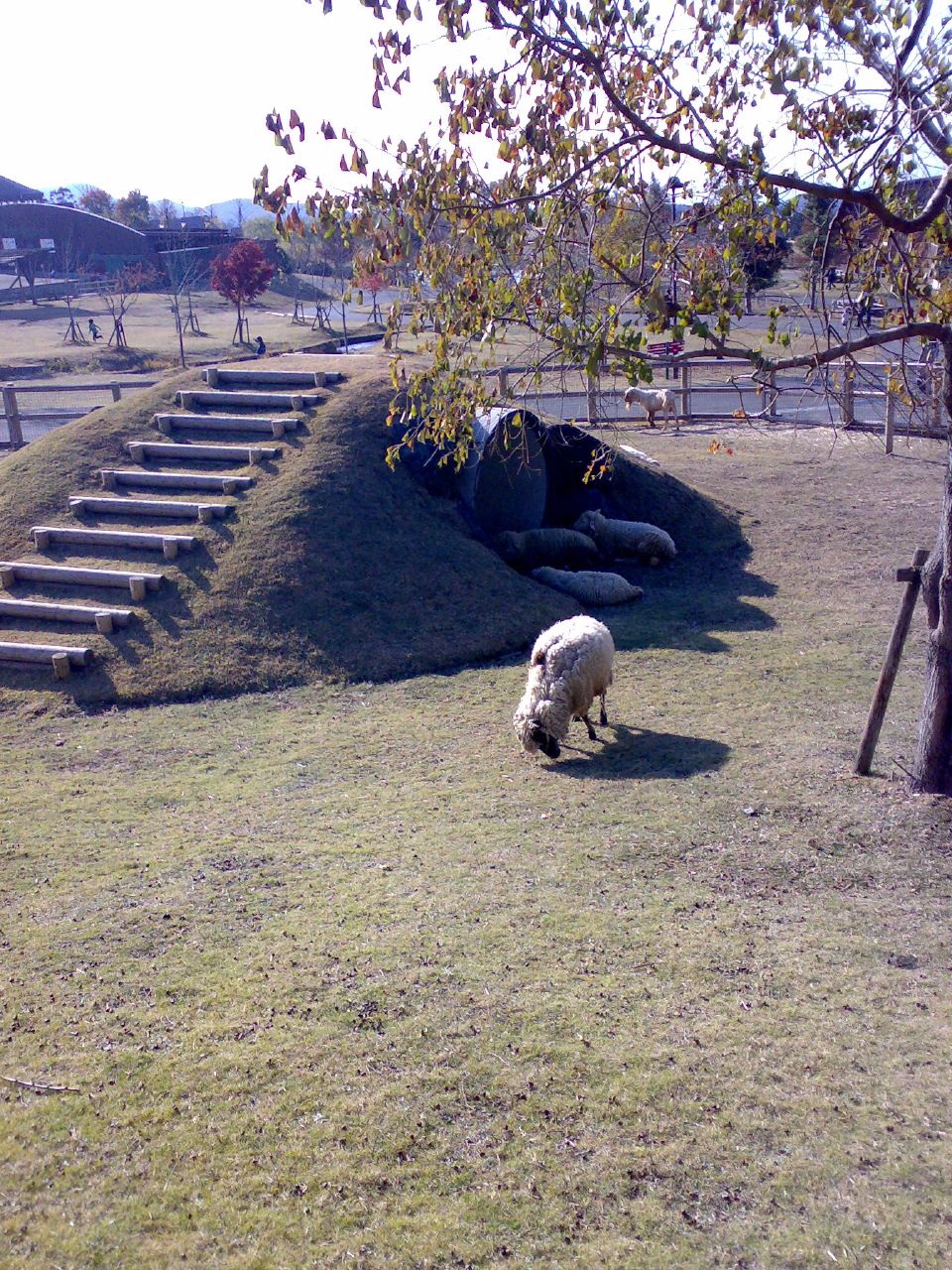The image depicts a lively scene at a petting zoo, featuring a well-maintained sheep pen. Dominating the foreground, a woolly white sheep with black feet and a black face is seen bending down to graze on the lush green grass. To the rear of this grazing sheep, a small grassy knoll rises, topped with wooden steps to prevent slipping during rain. Nestled under the hill, a large concrete cylinder, repurposed as a cozy sheep shelter, houses three more sheep resting at its entrance. The background reveals an enclosed area with a sturdy wooden railing, ensuring the sheep are safely contained. Amid the enclosure, stands a tree adorned with small leaves, adding a touch of natural beauty to the setting. Scattered around the pen, other sheep, including a less woolly shorn one, are either walking or lying on the grassy dirt terrain. The entire area is bordered by parkland and a road that snakes around the grassed zones, and two children can be seen in the distance, one of them running towards the left, adding a sense of liveliness and interaction to the peaceful pastoral scene.